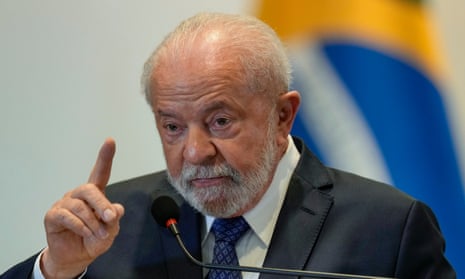In this detailed, close-up photographic portrait, an elderly white man is depicted indoors, head and shoulders visible. He appears to be in his 70s or 80s, with thinning grey hair and a white and grey beard and mustache. He's dressed meticulously in a grey suit with a white shirt and a blue tie adorned with white diamond patterns. His right hand is raised, with his forefinger pointing upward while the rest of his hand is clenched in a fist, suggesting he is making a significant point or emphasizing something during a speech.

His expression is serious, with a furrowed brow, and he is looking slightly down. His mouth is directed toward a black microphone that features a grey neck and a distinctive red collar. The clarity of the image highlights the man's well-manicured, short nails.

In the blurred background, there is a yellow object with blue and white bands, likely a flag, though it remains out of focus. The overall image is brightly lit, indicating ample natural light. The man's suit jacket has an opening for a pin, but no pin is present. There's no text in the image, ensuring the focus remains on the man's expressive gesture and serious demeanor.